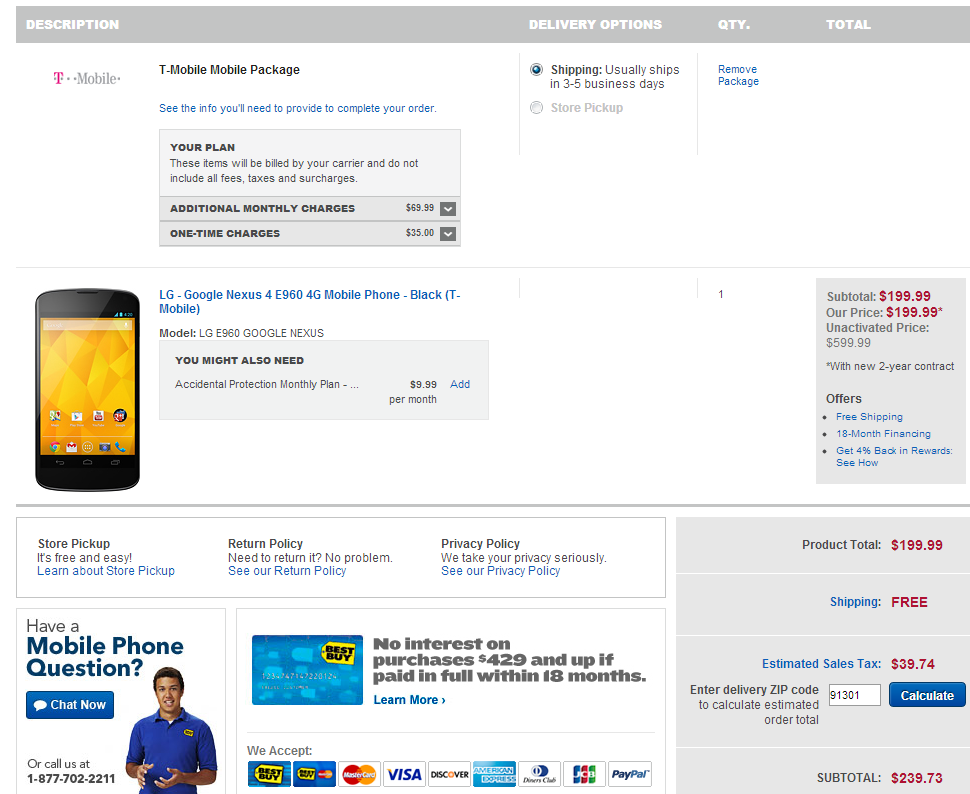The image depicts a detailed receipt from Best Buy for a mobile package from T-Mobile. The receipt outlines the necessary information for completing the order and specifies additional monthly charges of $69.99, along with a one-time charge of $35. The customer ordered the LG Google Nexus 4 E960 in black from T-Mobile, with the product model number clearly displayed. The receipt also suggests the optional accidental protection plan, which is available for $9.99 per month.

Shipping details indicate that the order is expected to arrive within three to five days, as the customer opted for shipping rather than store pickup. The package quantity is highlighted, and the subtotal for the order is prominently shown as $199.99 in red text. The unactivated price of the phone is $599 with a two-year contract, and the order includes offers such as free shipping, 18-month financing, and 4% back in rewards.

The receipt also provides information on the store pickup return policy and privacy policy. The product total is $199.99, with free shipping and an estimated sales tax of $39.74, bringing the grand total to $239.73 for the zip code 9301, which is also highlighted in red.

At the bottom of the receipt, there's an option to chat with a representative for any questions. This section includes an image of a Caucasian or tan-colored male wearing a Best Buy shirt. There's also a note about no interest on purchases of $429 and up if paid in full within 18 months. Accepted payment methods include Best Buy cards, Visa, MasterCard, Discover, American Express, and PayPal. The overall background of the receipt is primarily white with some gray-shaded areas, with important prices highlighted in red.